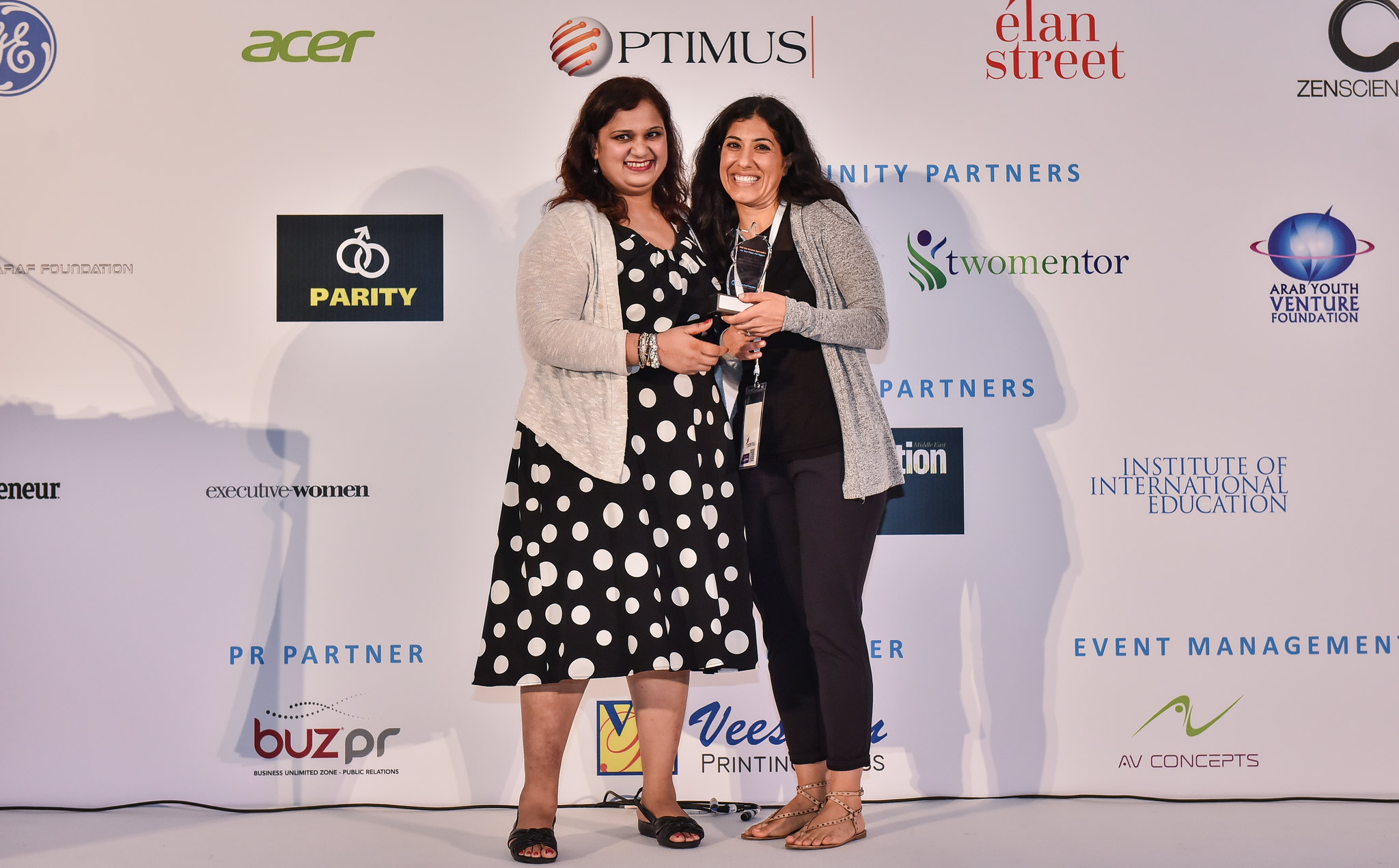In this rectangular photograph, two women are posing in front of a backdrop adorned with various sponsor and contributor logos, indicative of a convention or conference setting. The backdrop features recognizable names such as Acer, GE, Executive Women, Optimus, Elan Street, and the Institute of International Education, among others. The women, who appear to be of Middle Eastern or Asian descent, stand shoulder to shoulder, directly centered in the image, both smiling warmly at the camera.

The woman on the left is dressed in a black dress decorated with white polka dots, paired with a light gray open cardigan and a sparkly bracelet on her right wrist. Her companion on the right wears a black shirt with black leggings, a darker gray cardigan, sandals, and a lanyard around her neck, suggesting she might be an attendee or organizer. She holds a small white object, presenting it to the woman beside her. Both women have long black hair and darker skin tones. They are standing on a white podium or stage, enhancing the sense of formality and importance of the event.